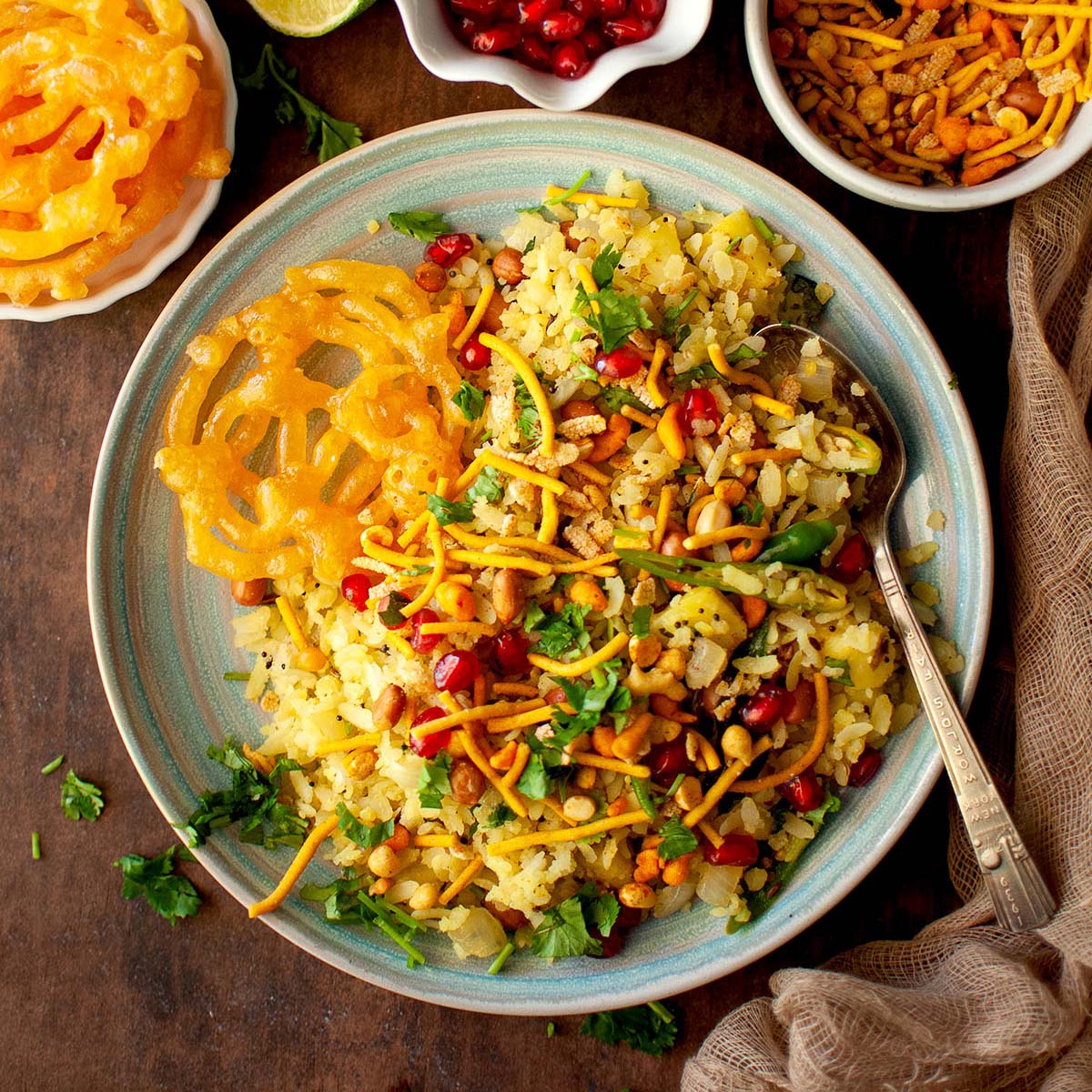This professionally taken, full-color photograph captures an overhead view of a meticulously arranged food scene, with no border and a vertically rectangular orientation. The primary focal point is a ceramic plate with concentric blue and brown circles, placed on a light to dark brown wooden table visible at the lower left and right corners. Scattered bits of seasoning resembling leaves are present on the table, adding a rustic touch. On the right side, a brown gauze napkin adds texture to the composition.

The plate itself features a medley of food, prominently showcasing a bed of rice mixed with smaller pieces of green cilantro or lettuce and red beans. Speckled among the rice are orange elements that appear to be fried onions, enhancing the dish's visual and textural appeal. A silver spoon rests on the right side within the plate, ready for serving.

In the upper section of the image, several bowls containing various accompaniments surround the main plate. At the upper middle sits a bowl of cranberries, while the upper right corner holds a mix of trail mix. The upper left corner presents an intriguing, woven, gelatinous yellow item that resembles a pretzel, whose exact nature remains unidentified. This detailed and vibrant composition suggests a healthy, wholesome meal, thoughtfully prepared and artfully presented.